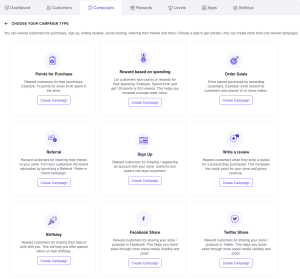The image is a cropped screenshot of a dashboard set against a solid white background. In the upper left corner, there is a label that reads "Dashboard." To the right of that are two other sections labeled "Customers" and "Campaigns." The word "Campaigns" is highlighted in blue text and is accompanied by a small icon to its left. Below, bold black text reads "Choose your campaign type."

There are three rows of options displayed, each with icons and buttons. The icons in the first row and the second row, although visible, are too small to read. However, in the third row, the center icon is identifiable as it reads "Facebook Share" with a Facebook icon positioned above it.